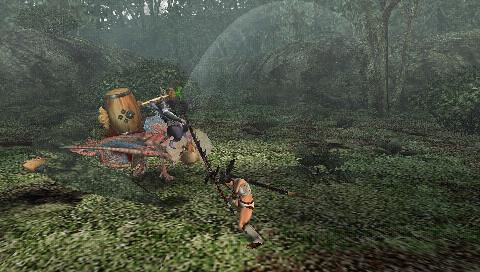This detailed color screenshot from an unknown video game captures a verdant, pixelated environment dominated by lush greenery, plants, and overarching trees. In the center, a player character stands prominently, appearing to interact with another character or animal to the top left. The latter is mounted on an animal-like figure, carrying a wooden cask or barrel on its back. The main character in the fore seems to be wielding a long sword, while the other is seated on a rocky structure, possibly engaged in some hauling activity involving a barrel. The entire scene brims with dense vegetation, including grass, bushes, and trees, creating an immersive wilderness backdrop. There are no buildings, motorized vehicles, or textual elements in the image, emphasizing the natural, untamed setting of this mysterious game.